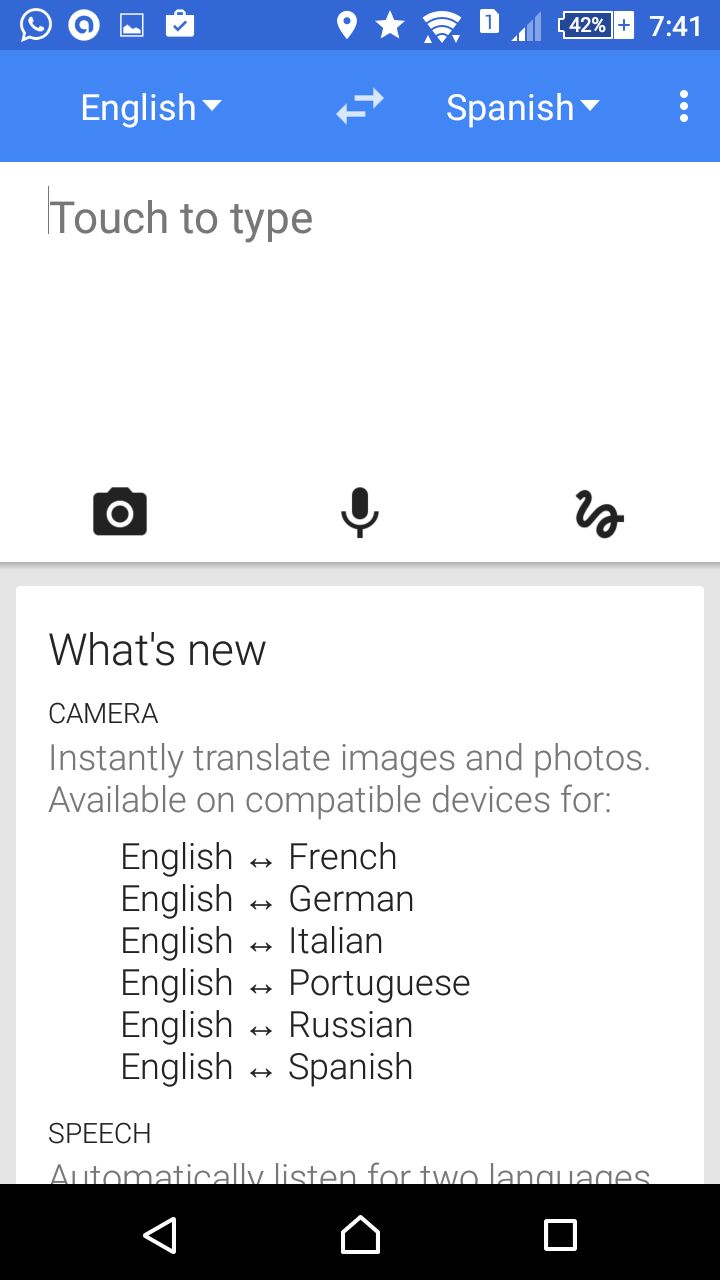Screenshot of the Google Translate App:

At the top of the screenshot, various status icons are visible: a location icon, a star, Wi-Fi signal, network bars, and a battery indicator showing 42% charge. The current time is displayed as 7:41. To the right of these icons, there are several app icons: WhatsApp, an app labeled "Ali," a gallery or picture app, and what appears to be a shopping bag with an arrow inside it.

Below the status bar, the Google Translate interface shows translation settings from English to Spanish. Two arrows point in opposite directions, indicating the translation direction. A text input field prompts "Touch to type," accompanied by icons for camera, microphone, and handwriting input (represented by a squiggly line).

A notification box below the input field highlights new features, mentioning that the app's camera can now instantly translate images and photos for certain languages directly on the device.